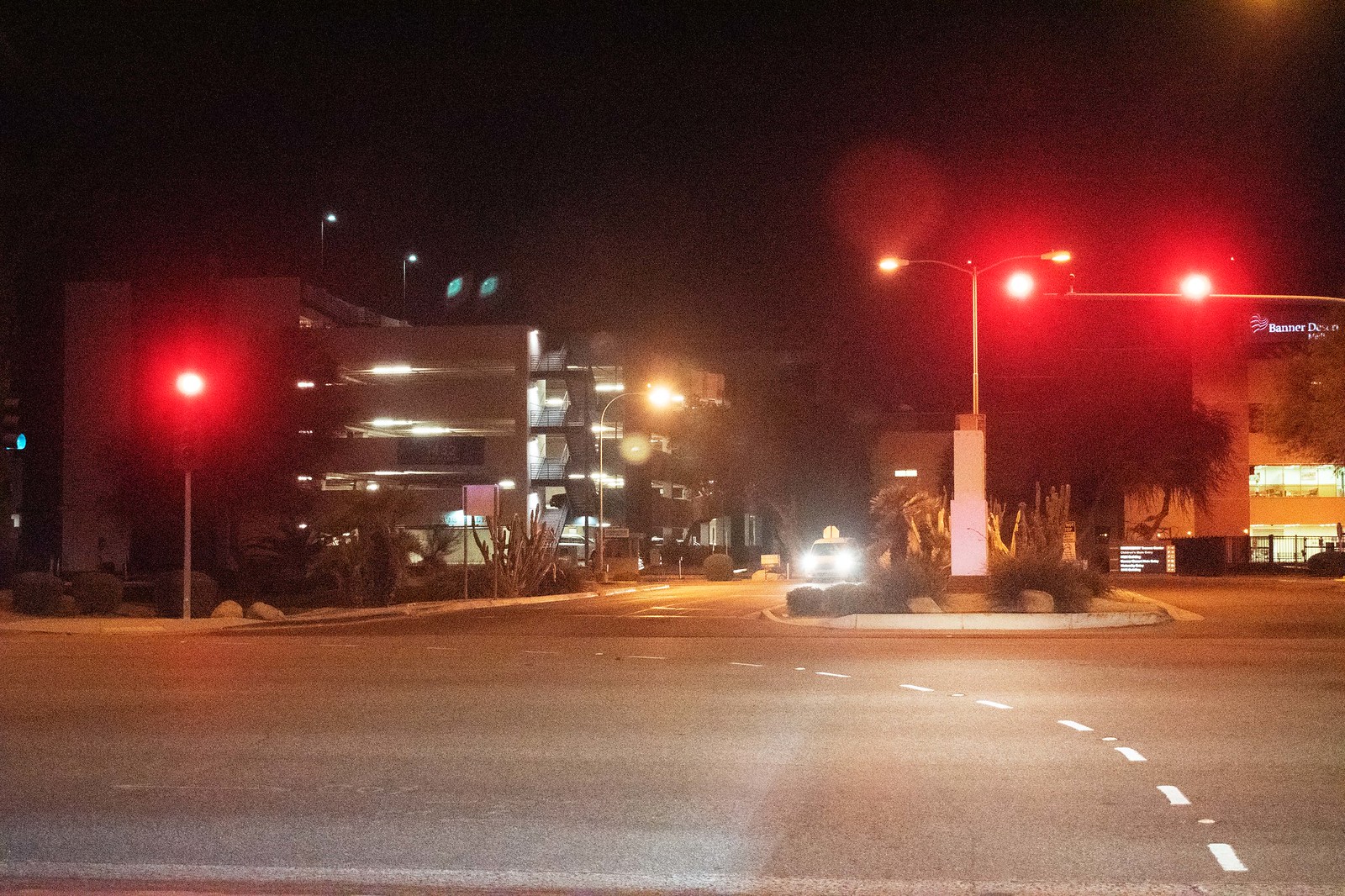The image depicts a nighttime urban street scene with a dark night sky overhead. The roadway is composed of gray asphalt, marked with white dotted lines that delineate a turn lane. In the foreground, three red traffic lights can be seen — two on the right side and one on the left. Centered in the image, a tall street sign is situated on a small landscaped island bordered by a curb. This island boasts several bushes and taller plants, contributing to the greenery.

Prominently rising from the island is a tall white rectangular lamp post. At its base is a cylindrical structure from which extends a long rod with two lamps on either side.

In the background to the left, a large white building is noticeable, featuring what seems to be a multi-story parking garage with four or perhaps five floors, including the roof. The structure includes a staircase encased in glass windows, revealing its floors from top to bottom. On the right side of the image, another white building with a square-like shape rises up, comprising two or three stories. At its top, a white banner with text adorns the building, though the specific wording is indiscernible.